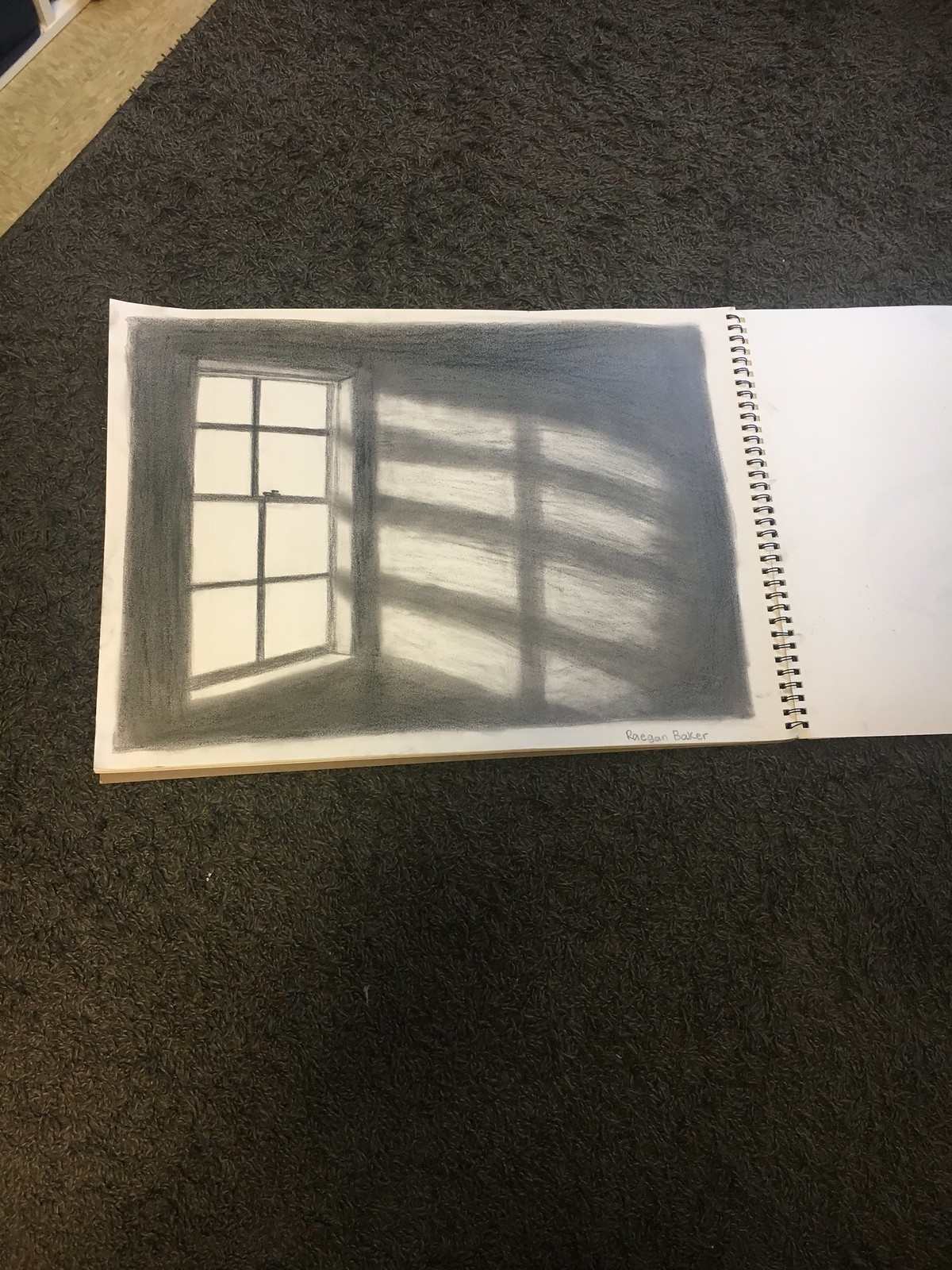A meticulously detailed pencil sketch depicts a window divided into eight sections by crossbars, allowing light to pour through and form intricate shadows on a nearby wall. The sketch is drawn on a white, open notebook with silver rings binding the pages together at the center. Placed on a textured, carpet-like black surface, the notebook lies flat as the camera captures it from a top-down perspective, emphasizing the contrast between the light and shadows in the artwork. The monochromatic palette of the drawing accentuates the interplay of light and dark, creating a visually striking effect.